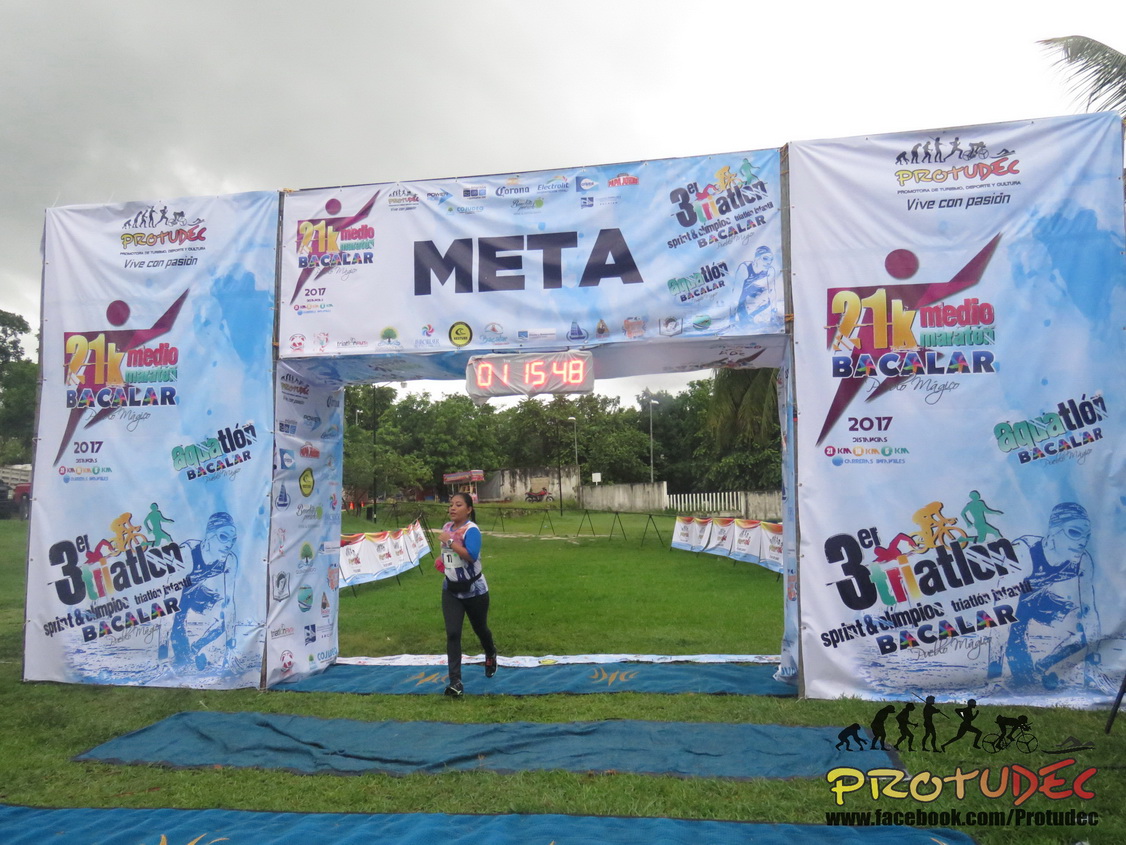In this image, a woman is captured running through the finish line of a marathon event. She is dressed in black leggings, a white and blue shirt, and a black fanny pack around her waist. Pinned to her shirt is a race number. The scene is set on a grassy area adorned with several trees. Overhead, a large archway marks the finish line, prominently displaying a timer that reads "01:15:48" in red digits. Inscribed on the archway is "META," and to its left, in colorful text, it reads "21K Media Maratón Bacalar." The background reveals an overcast sky, with gray clouds on the top left and lighter clouds on the top right. Additionally, there is a yellow and red watermark at the bottom right that reads "PROTUDEC" followed by a black Facebook URL, www.facebook.com/protudeck. The surrounding area features signs and fences, contributing to the organized setup of this outdoor event.